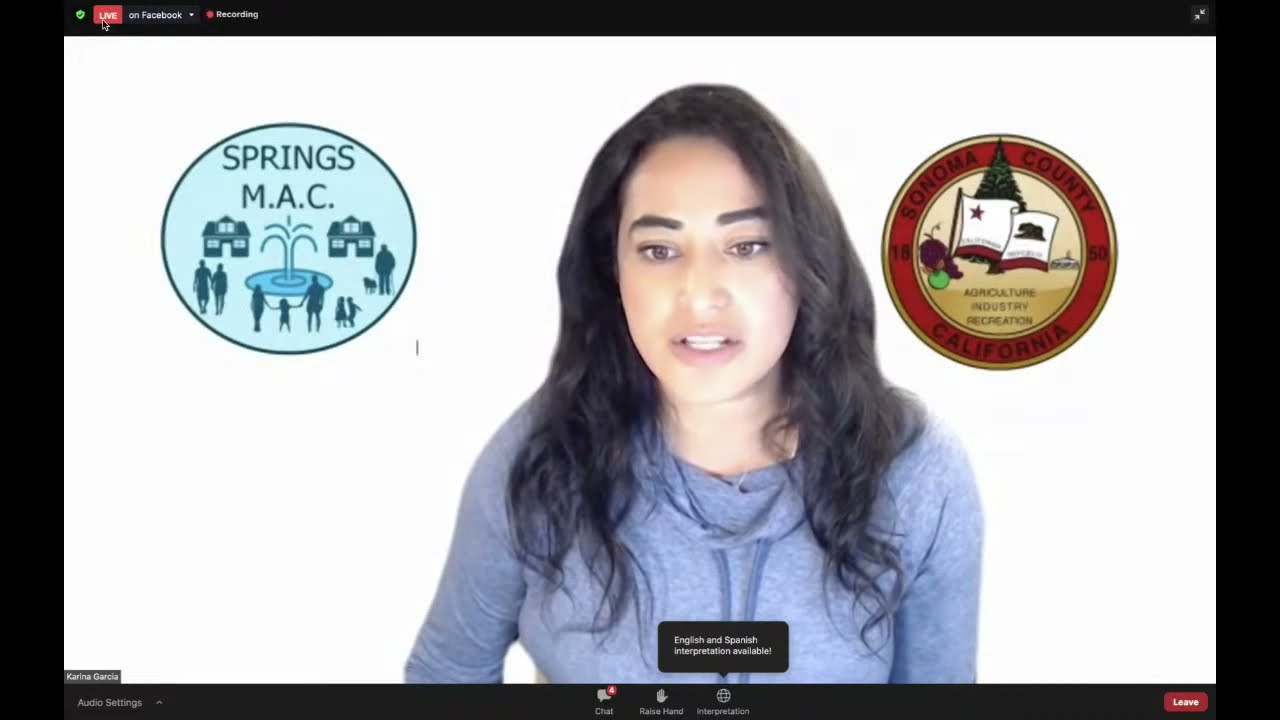The image is a webcam capture from a video conferencing platform, resembling a Zoom meeting, with thin black bars framing the video on the left and right. It features a young woman with dark, flowing hair, dressed in a blue hoodie with visible strings, against a white background. On the top left corner, there is a red "live" button with the text "on Facebook" and a recording button beside it. The bottom bar displays various icons including audio settings and a leave button on the left and right, respectively, with a chat icon underneath.

Positioned over her right shoulder (viewer's left) is a blue circular emblem with text "Springs M.A.C." at the top and a design featuring a central fountain surrounded by several figures: a couple, a family, and a man with a dog. The emblem also includes two houses. 

Over her left shoulder (viewer's right) is the Sonoma County, California emblem. This emblem is a circular seal with a maroon or brown outer band containing the words "Sonoma County, California," and a tan-colored inner circle. The inner circle depicts the California state flag with a star and bear, set against a backdrop of a pine tree, and includes the motto "Agriculture, Industry, and Recreation" at the bottom.